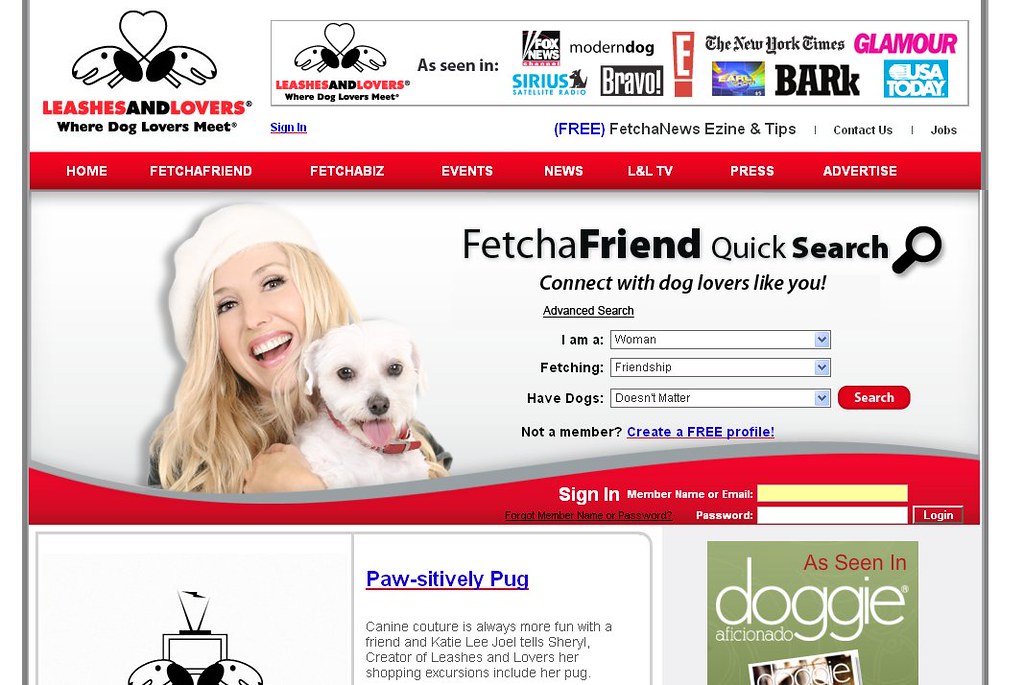This is a screenshot of an outdated website, possibly from several years ago. In the upper left-hand corner, there's a peculiar logo depicting two dogs looking to the side, connected by a heart. Below the logo, red text reads "Leashes," followed by "Lovers" in black text and "Where Dog Lovers Meet" in black further down. Adjacent to the logo is a large rectangular section that repeats this text and includes the phrase "As Seen In," followed by logos for various media outlets including Fox News, Sirius Satellite Radio, Modern Dog, Bravo, E!, The New York Times, Glamour, USA Today, and Bark.

Below this section is a red navigation bar featuring links labeled "Home," "Fetch a Friend," "Fetch a Biz," "Events," "News," "LNL TV," "Press," and "Advertise." Further down, there's an image of a smiling blonde woman wearing a white beret and holding a white dog. 

Next to this image, there is a "Fetch a Friend Quick Search" feature with a magnifying glass icon and the tagline "Connect with dog lovers like you." The interface includes options for an advanced search. The search section contains options for specifying that "I am a woman fetching friendship," with an additional field indicating that having dogs does not matter, followed by a search button. The design and elements suggest that the website is quite old and outdated.